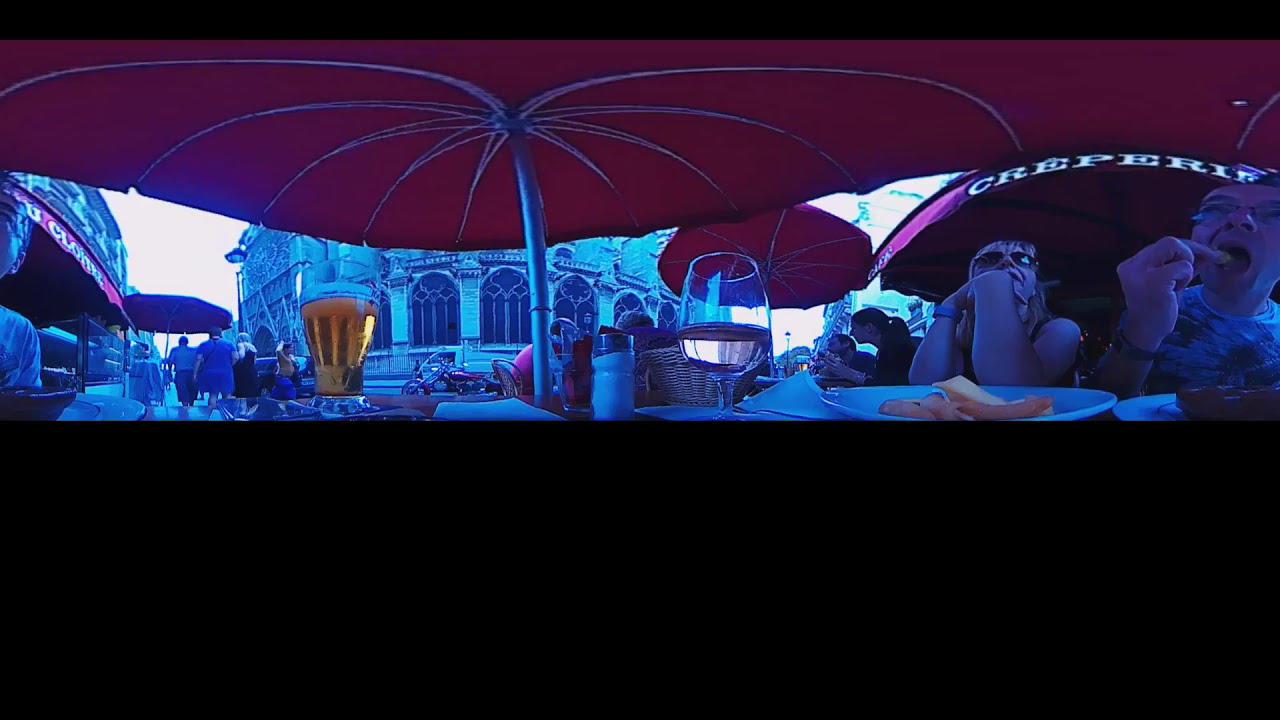In an eerily blue-tinted photograph of a European city at twilight, people are seated under red umbrellas at a sidewalk café. The scene features detailed architectural elements such as arched windows on a concrete building in the background. Central to the image is a couple on the right: an older man wearing glasses, caught in the act of eating, and a woman in sunglasses. The table in front of them holds a glass of beer, a glass of wine, a salt shaker, and some hors d'oeuvres. Additional people populate the café, while the name "Creperie" is visible on the far-right red canopy. The surrounding elements add to the picture's charm with another smaller umbrella in the distance and an alleyway suggesting a pedestrian-friendly environment. The overall ambiance has an almost surreal quality due to the color manipulation, with vivid reds and cool blues dominating the scene.